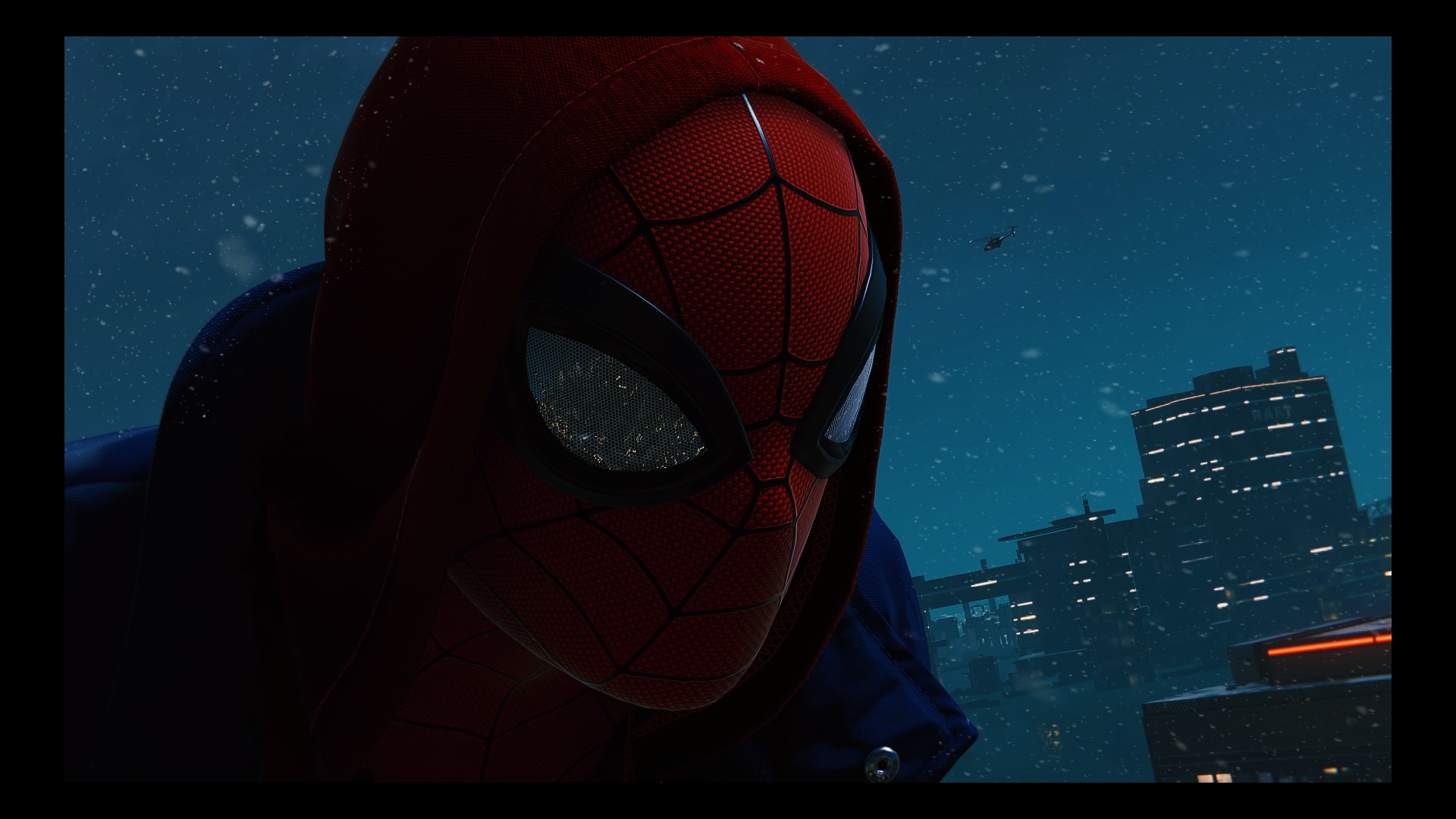This computer-generated graphic portrays a close-up of Spider-Man against a twilight or early evening skyline. Positioned slightly to the left, Spider-Man’s upper torso and head are featured prominently. He dons his iconic red mask adorned with black spider web patterns and distinctive silver eyes outlined in thick black bands. His attire includes a red hoodie over his head and an open navy blue puffer jacket, implying a sense of concealment or an attempt to keep warm. Behind him, the dark blue, star-speckled sky accentuates the urban backdrop to the right, filled with illuminated skyscrapers. One noticeable building near the lower right has an orange strip of light across its rooftop, adding a unique burst of color. The entire graphic is outlined in black, enhancing its distinct contours and elements, including a small black silhouette in the sky, possibly suggesting a hovering helicopter.